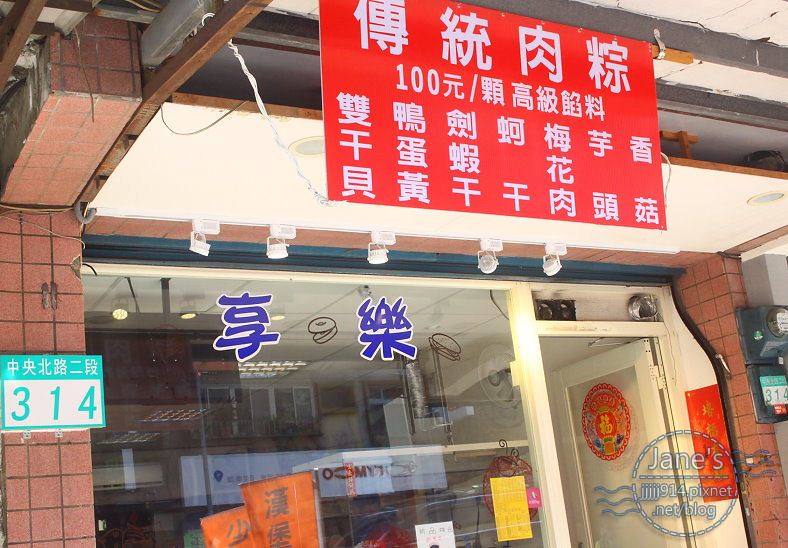The image depicts the storefront of a Chinese restaurant, characterized by a prominent red and white sign featuring Chinese characters. The building itself is constructed of red brick or brick-colored tiles, and the front of the store is dominated by large glass windows. Through these windows, one can see various items inside, illuminated by interior lighting. A white door, framed by white wood, stands open, displaying blue Chinese character decals on either side. 

Above the storefront hangs a red banner with white symbols, including the number 100 and additional Chinese characters. Also visible on the door is a red seal or crest. Just to the left of the door, painted on the glass, are outline images of a sandwich and a bagel. An address sign on the side of the building reads "314" in blue, with white Chinese characters above it. 

In the reflection of the store's glass windows, another storefront with a white awning and multiple lights can be seen across the street. The entire scene is brightly lit by daylight, emphasizing the vibrant colors and detailed features of the restaurant's exterior.